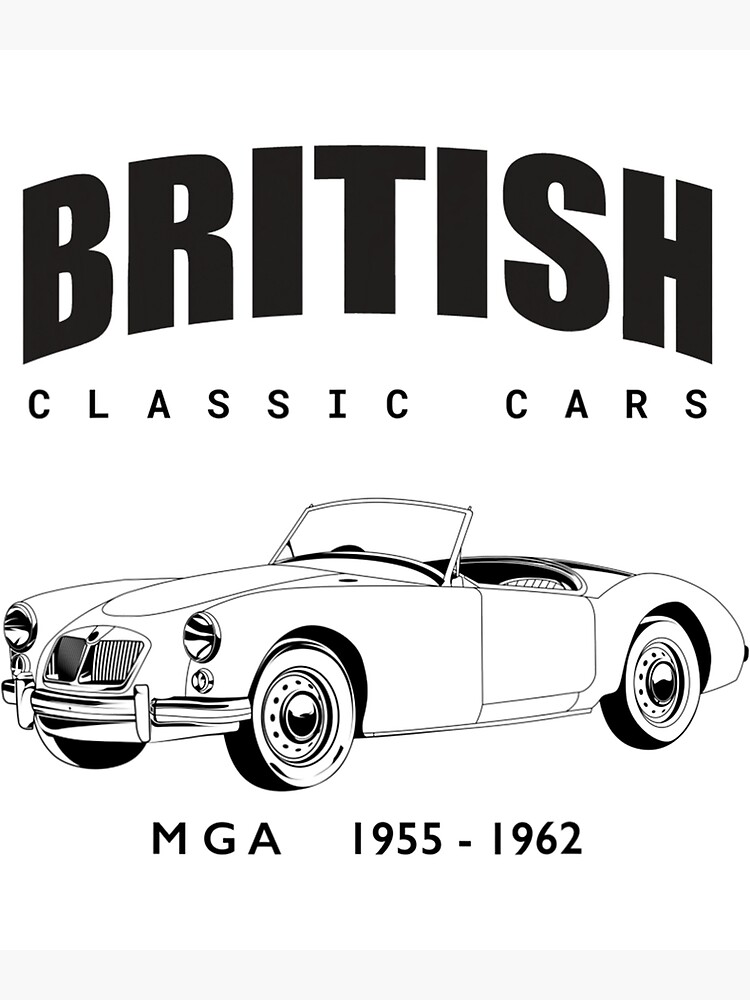This advertisement features a striking black-and-white illustration of a classic convertible car. In bold, large, all-caps black text at the top, it reads "BRITISH," and just below, in slightly smaller black text, "CLASSIC CARS." Below the image, it states "MGA 1955-1962." The vehicle depicted is a sleek, hoodless model from the 1950s or 1960s, showcasing elegant curves around the hood and trunk, and it is rendered with a delicate balance of thin outline drawing and detailed elements such as its standard-style wheels, headlights, and small, fancy grille. The car is viewed at an angle, highlighting its rectangular windscreen and just revealing the top edge of the seats inside. The entire scene is set against a clean, white background, emphasizing the timeless beauty of the classic British automobile.